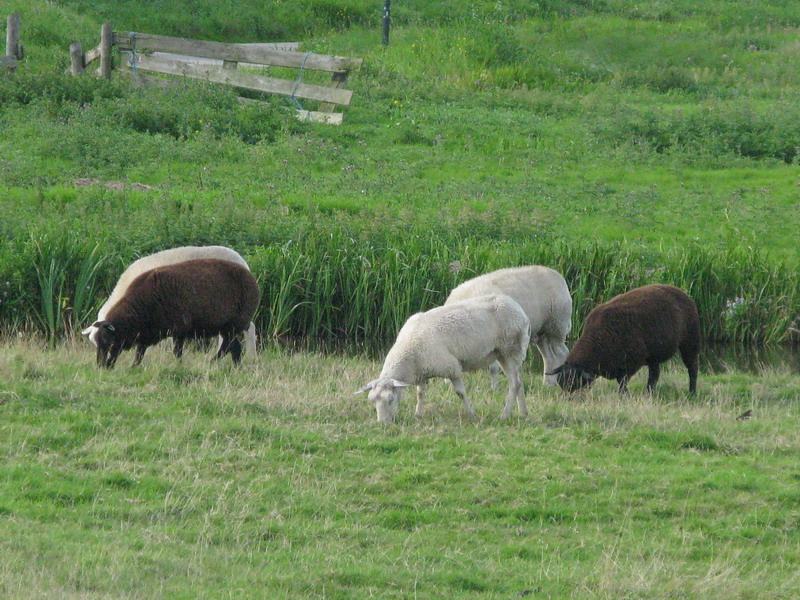A vibrant, expansive field of long grass, possibly used for hay, spreads across the image, with green metal poles hinting at a barely visible wire fencing in the distance. Toward the upper left, an old, decrepit wooden wagon adds a rustic charm. In the middle of the image, where the tall grasses have been cut down, five adorable, fluffy sheep are grazing. Three of them are white and two are black, though the sun has tinted their wool a brownish hue. Their wool, appearing to have regrown for a couple of months post-shearing, gives them a cute, somewhat fluffy appearance. The sheep are contentedly munching on the shorter, vibrant green grass amidst patches of dry, beige blades. Behind them, taller grass signifies untouched growth. An aged, weathered wooden fence and gate, bearing dark brown or black accents from exposure, lingers in the background. The scene is sunlit, casting reflections and highlighting the contentment of the sheep in their serene, pastoral setting.